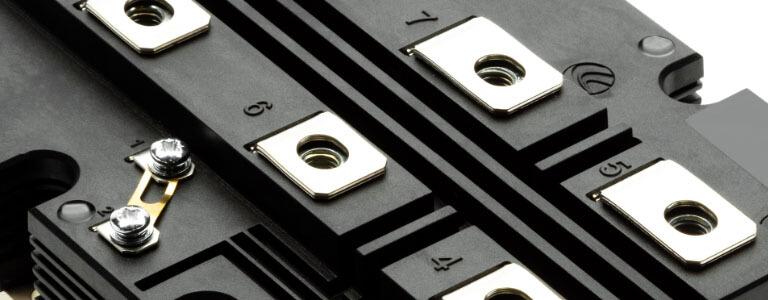This image depicts a close-up of a black panel or possibly a bracket, exhibiting a matte black finish with both plastic and metallic elements. The panel features numbers engraved on its surface—specifically 4, 6, 7, and 5—which seem to correspond to nearby holes, likely for rivets or screws. These numerical markers and holes suggest a structured layout, typical of mechanical or electronic components. The top part of the panel shows a series of slats resembling vents, and the bottom left corner contains two shiny, metallic screws arranged diagonally and connected by a gasket-like element. There is also a small metallic, possibly copper, shiny piece near these screws. The panel seems designed for mounting or securing within a larger assembly, such as electronic equipment. The detailed craftsmanship, including the combination of matte and polished finishes, highlights its purposeful engineering.